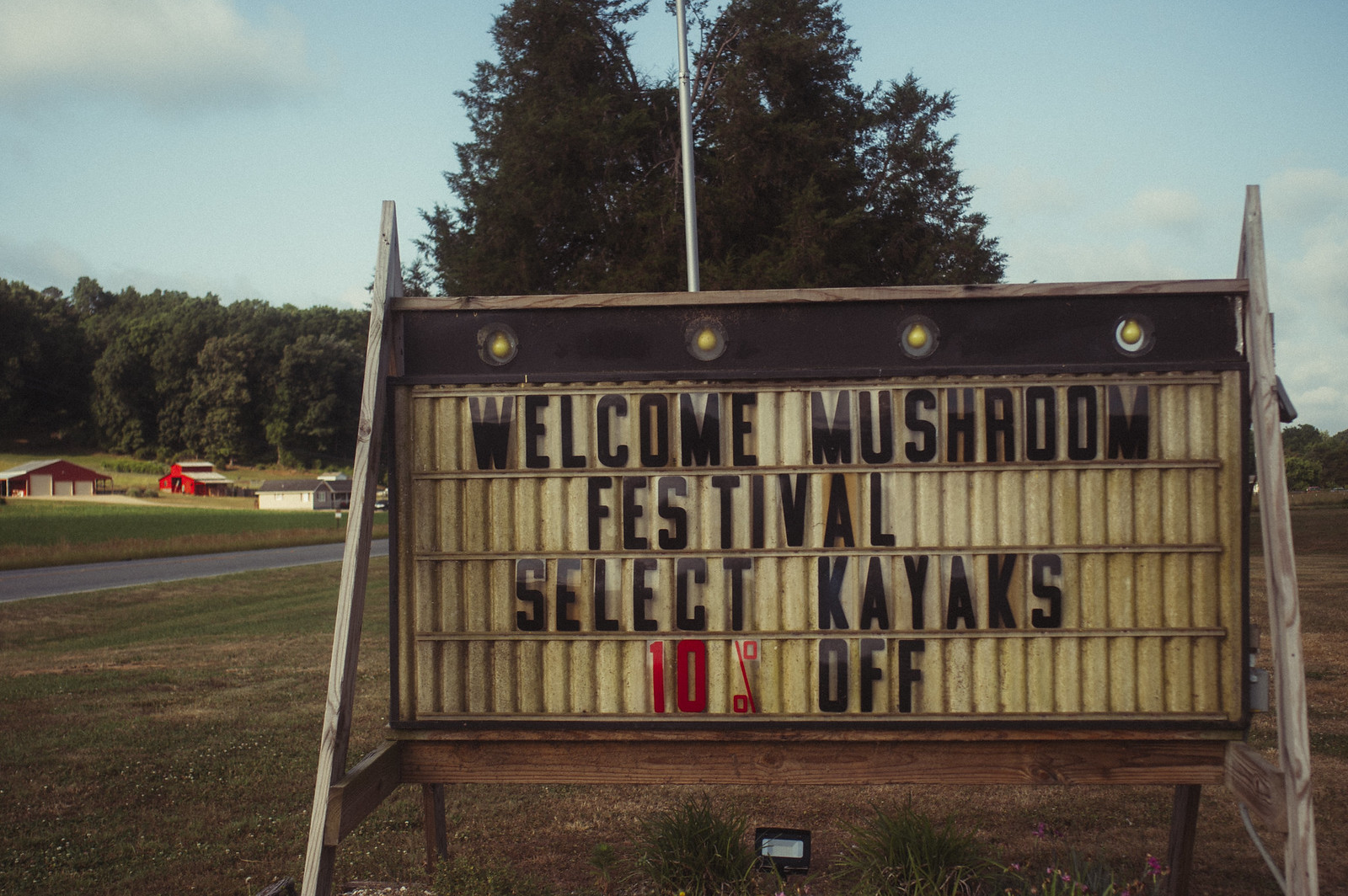This photograph captures an outdoor marquee sign, rectangular in shape with a distinctive black top border embellished by four yellow bulbs. The sign prominently displays the message: "Welcome Mushroom Festival. Select kayaks 10% off." Here, the number "10" and the percentage sign are strikingly rendered in red, contrasting with the rest of the text in black. The sign is illuminated by a spotlight positioned in front of it. The surrounding area appears sparse, with patches of grass and a couple of low bushes beneath the sign. The scene is bathed in daylight, with a vividly blue sky overhead, dotted by a few fluffy white clouds.